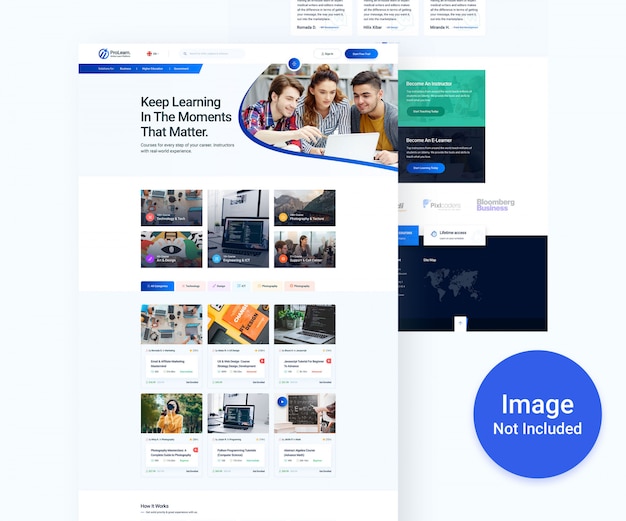The image features a gray header at the top, containing three indistinct white boxes with illegible text due to lack of focus. Below the gray header, there's a main screen with a button situated at the upper right corner. Directly below this button is a dark blue menu bar displaying the text, "Keep learning in the moments that matter."

To the right of this menu bar, a photograph depicts three individuals gathered around a laptop computer on a table or desk. The person on the left is wearing a blue and red plaid shirt, the woman in the middle is dressed in a white and black striped shirt, and the person on the right sports a brown shirt with a gray shirt layered over it.

Beneath the photograph, there are twelve uniformly arranged boxes, organized into four rows of three. On the far right side of the image, a light blue circle contains the text "Image not included."